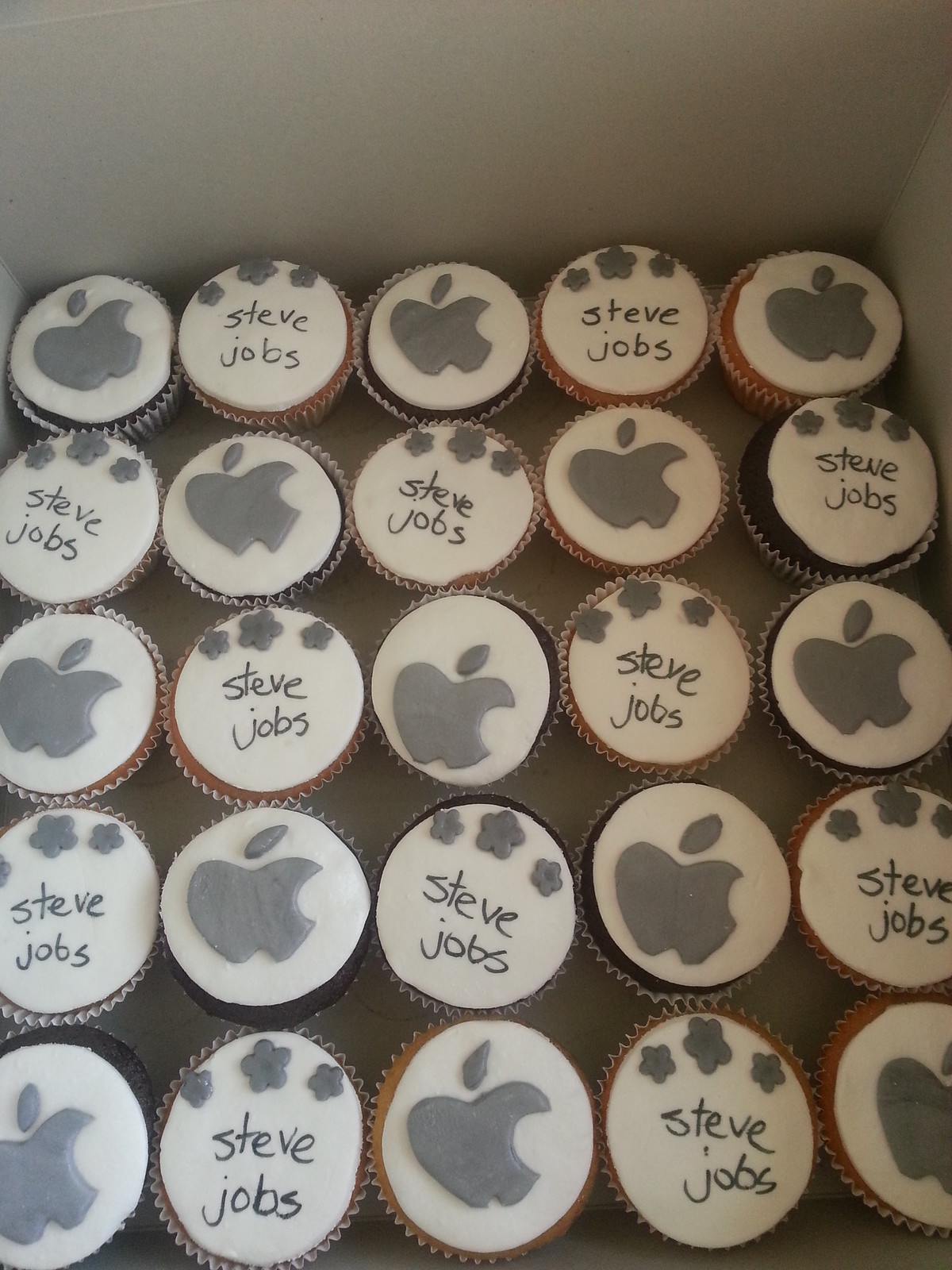This image is a tall, rectangular photograph showcasing a box of 25 cupcakes arranged in five rows of five. The box, which is of a light gray or off-white color, has its top edge partially visible. Each cupcake alternates between chocolate and vanilla bases. The cupcakes are topped with white circular icing and have two different designs: some are decorated with the Apple logo made from gray frosting, which features a little leaf and a circle cut out of the right side, while the others have three small five-petaled flowers, also in gray frosting, with the name "Steve Jobs" written underneath. The cupcakes, despite their uniformity in pattern and design, show minor variations typical of being handmade.